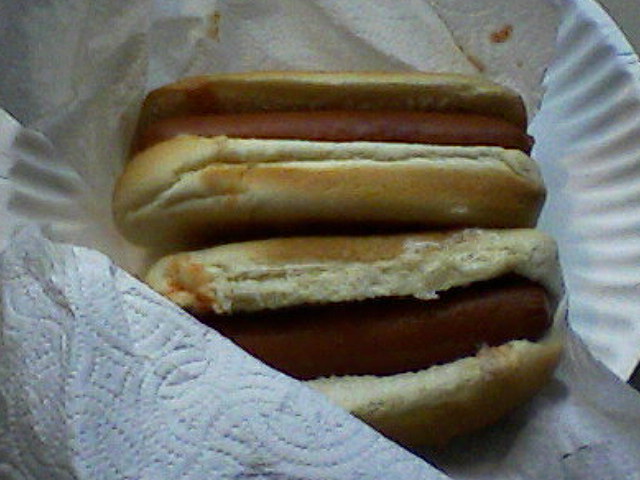The photograph showcases two hot dogs, each nestled in a split, bun-length bun, devoid of any toppings or condiments. These hot dogs rest on a brown paper towel, which itself is positioned on a flimsy white paper plate, identifiable by its pleated edges. Notably, the brown paper towel curves upward at the bottom, slightly wrapping over the edge of one of the hot dogs, which contributes to a clear view of the scene. Dark stains, possibly remnants of ketchup, mark the brown paper towel. Additionally, a white quilted paper towel is visible in the lower left corner of the image, contrasting with the brown paper towel and white paper plate. The background reveals part of a white tabletop in the upper right corner. This minimalist setting emphasizes the simplicity of the hot dogs and their surroundings.